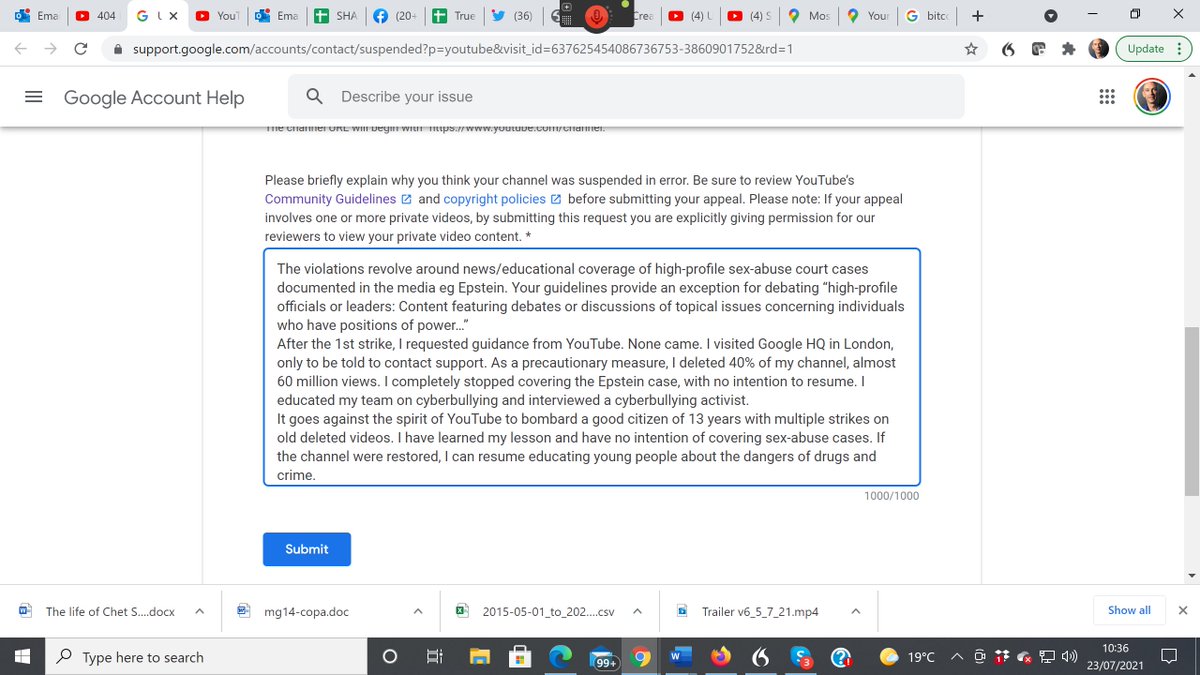This screenshot features a cluttered computer screen, indicative of a busy individual. The taskbar at the bottom reveals numerous open applications, alongside a Google Chrome window with multiple tabs in use. The focal point of the screenshot is a detailed and impassioned appeal on a Google Account Help Support page. The user has typed a long message addressing an issue concerning violations related to news and educational coverage of high-profile sex abuse court cases, specifically mentioning the Epstein case. They discuss the exceptions within YouTube's guidelines for debated content featuring individuals in positions of power. The message details the user's proactive steps following a first strike, including visiting Google HQ in London, deleting 40% of their channel content amounting to almost 60 million views, and ceasing coverage on the Epstein case. They also mention efforts to educate their team on cyberbullying and their interviews with cyberbullying activists. The appeal emotionally argues that over 13 years on the platform, the user has learned their lesson and seeks the restoration of their channel to continue educational efforts on the dangers of drugs and crime. A "Submit" button is ready to be clicked, underscoring the user's hope for resolution and reinstatement.